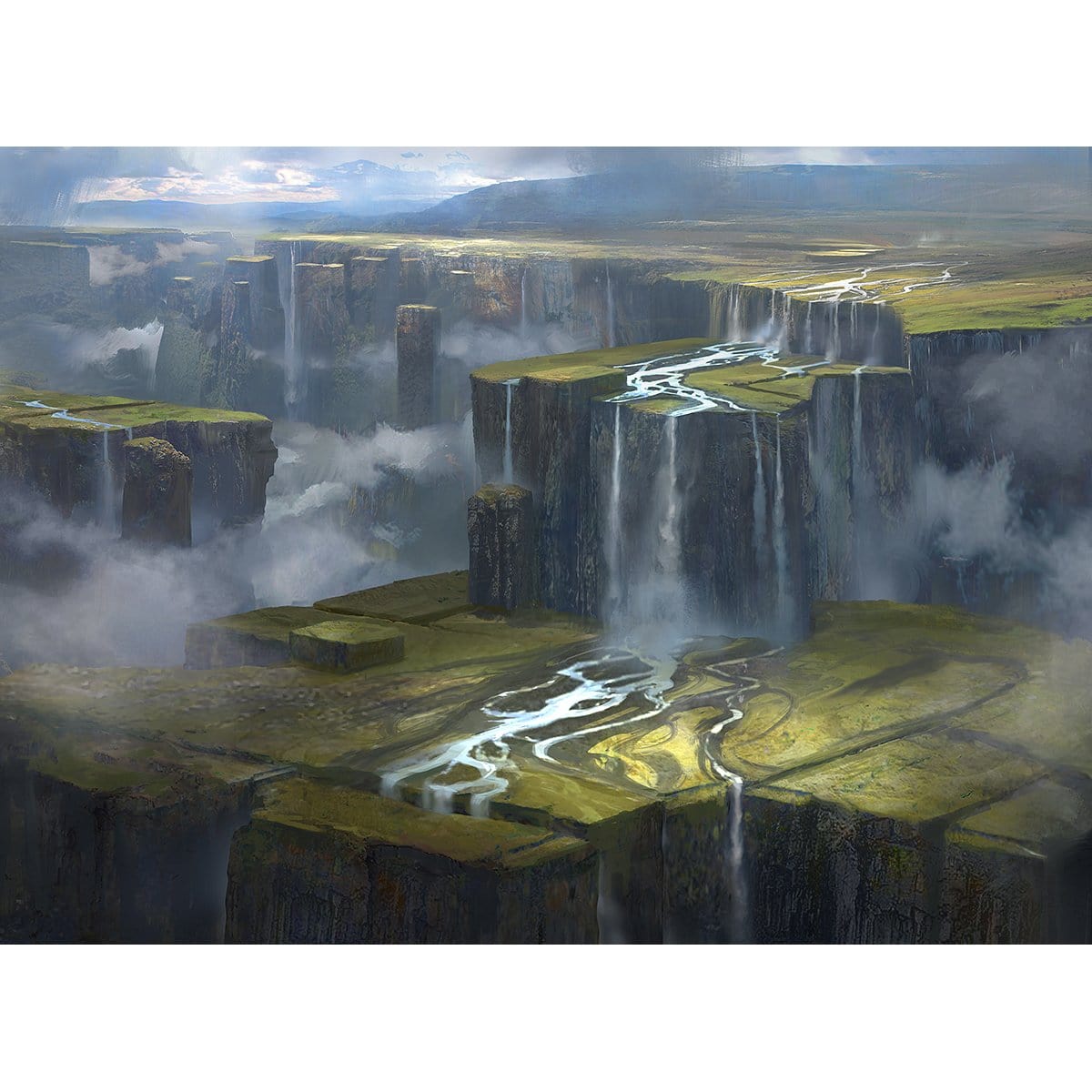The painting showcases an imaginative and surreal landscape of multi-tiered plateaus that resemble sliced blocks of earth. The land is segmented into various squares and rectangles, with flat, green tops and steep, vertical earth-toned sides. From the top right corner, a river meanders through the scene, transforming into waterfalls that cascade dramatically from one plateau to the next. Wispy clouds and dense mist envelop the scene, likely generated by the numerous waterfalls and the elevation disparities. In the distance, a gray-colored mountain rises behind the highest plateau, set against a vibrant blue sky adorned with large white clouds. The light in the painting appears to emanate from the top left, casting subtle shadows across the fantastical terrain. This elaborate depiction evokes a sense of a mystical, otherworldly landscape, akin to the dramatic cliffs found in places like New Zealand, yet distinctly surreal in its execution.